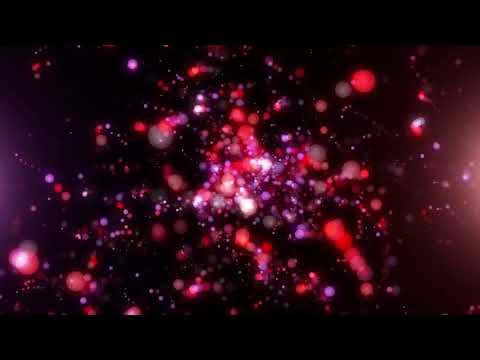The image is an abstract scene framed by horizontal black bars at the top and bottom, reminiscent of a cinematic aspect ratio. Against a predominantly black background, a dazzling array of red and purple lights are scattered throughout. These lights are clustered densely in the center, giving the impression of a galaxy formation, though not perfectly structured, and they disperse more sparsely as they move outward. Among these lights, some appear closer and blurry while others seem distant. Additionally, there are subtle glows enhancing the edges, with a reddish hue on the right and a bluish tint on the left. The image evokes a sense of glitter tossed into the air, with the lights sparkling and emanating in various directions as if captured mid-motion, creating a beautiful and mesmerizing display.